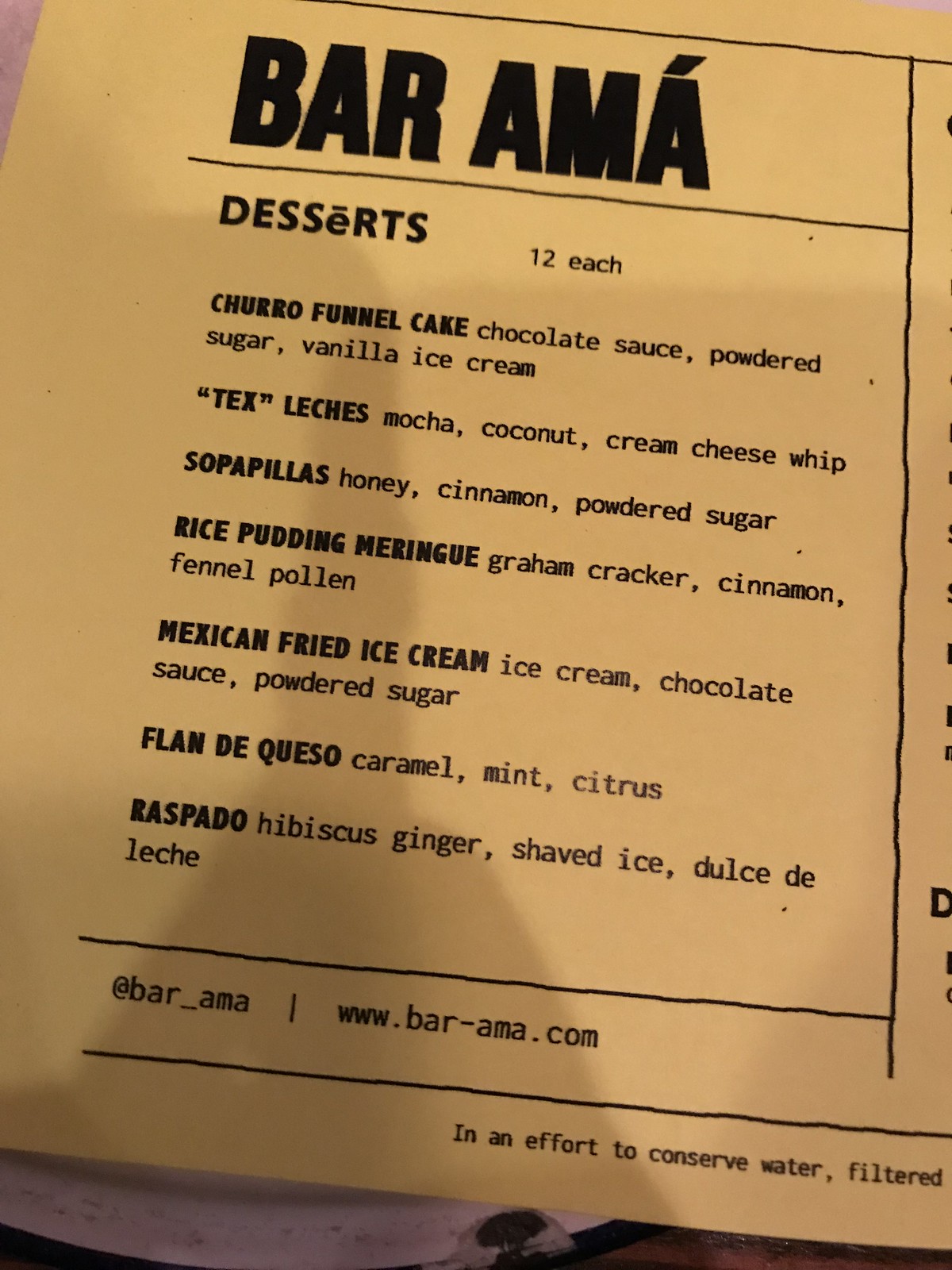This image displays a menu from a Hispanic or Mexican food restaurant. The menu has a yellowish-brown background that provides a warm and inviting feel. At the top, in bold black text, the name "Bar'ama" is prominently displayed, with a noticeable apostrophe above the "A."

The dessert section is detailed and mouth-watering, featuring an array of offerings including:
- "Flan de Queso" (Cheese Flan)
- Caramel
- Mint
- Citrus
- Respadó
- Hibiscus
- Ginger
- Shaved Ice
- Dulce de Leche

At the bottom of the menu, additional details are provided in a clear, concise manner. The Instagram handle "@bar_AMA" is listed along with their website "www.barama.com." A note at the very bottom reads, "In an effort to conserve water, filtered water is served upon request," emphasizing the restaurant's commitment to sustainability.